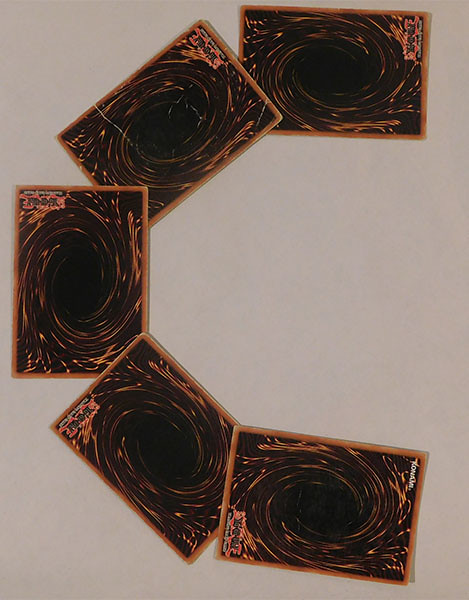The image showcases a set of five trading cards, possibly Yu-Gi-Oh! cards, each featuring a consistent design and size. The cards display a distinctive logo in red, with black and white text beneath it that is not legible. The backdrop of each card is black, adorned with coppery, orange-red swirls that create an electric, vortex-like effect, reminiscent of a black hole. These cards are arranged on what looks like a cream-colored table or background, positioned in a C-shaped formation. The first card is placed at the top right, with each subsequent card touching the bottom left corner of the previous one, creating a cascading effect that culminates with the last card nearly vertical on the left side of the image. The arrangement gives a sense of motion and dynamic visual interest.